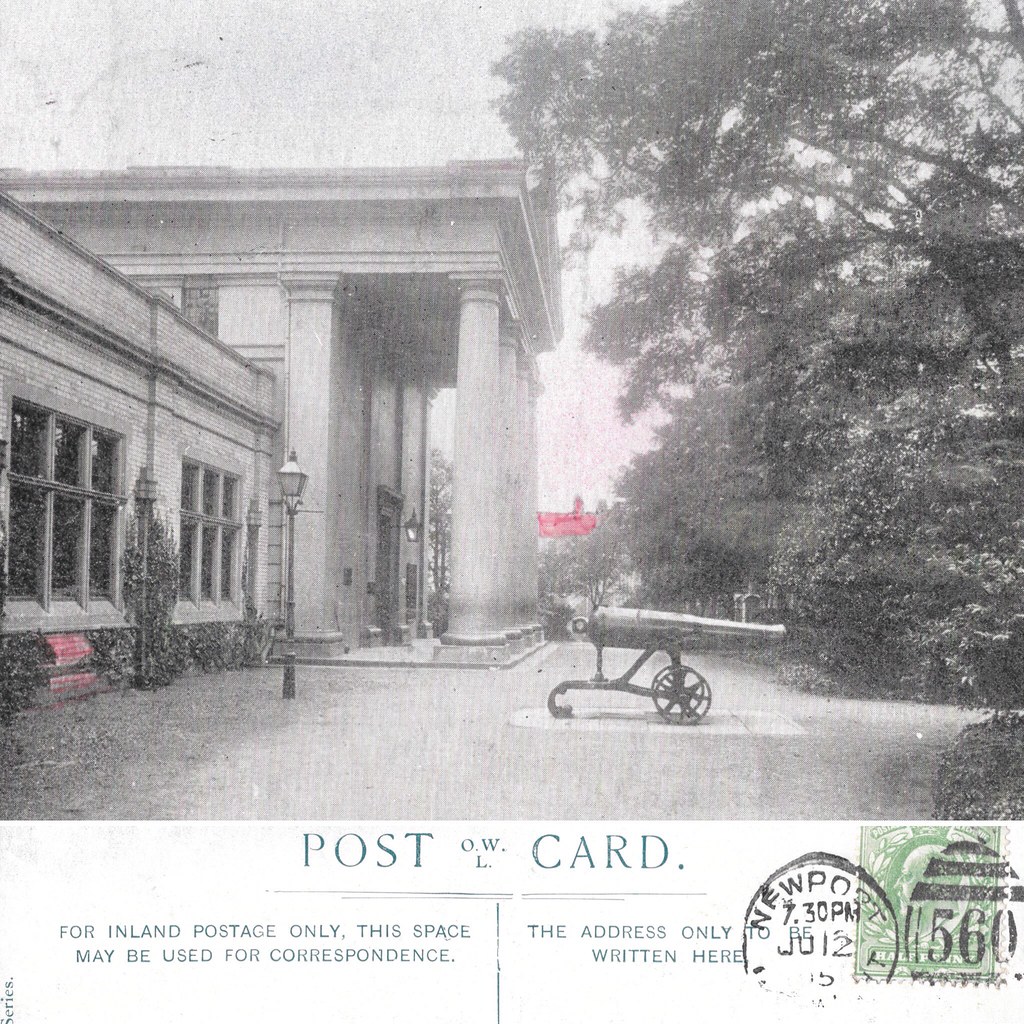This black-and-white vintage postcard features a grand stone building with four prominent columns at its entrance and large windows on either side. The building is adorned with old-style outdoor lighting and sits alongside a sizeable old-fashioned cannon mounted on wagon wheels, likely for decorative purposes. To the right of the building, several tall trees provide a picturesque backdrop. 

The bottom of the postcard is marked with the words "post OWL" in the center, and "card" on the right. Additionally, there's a section labeled "for inland postage only, this space may be used for correspondence," followed by "the address only written here." The postcard bears two stamps: one from Newport dated July 12th and another with the number 560. There are signs of red or pink coloring, which appear to be stains on the image.